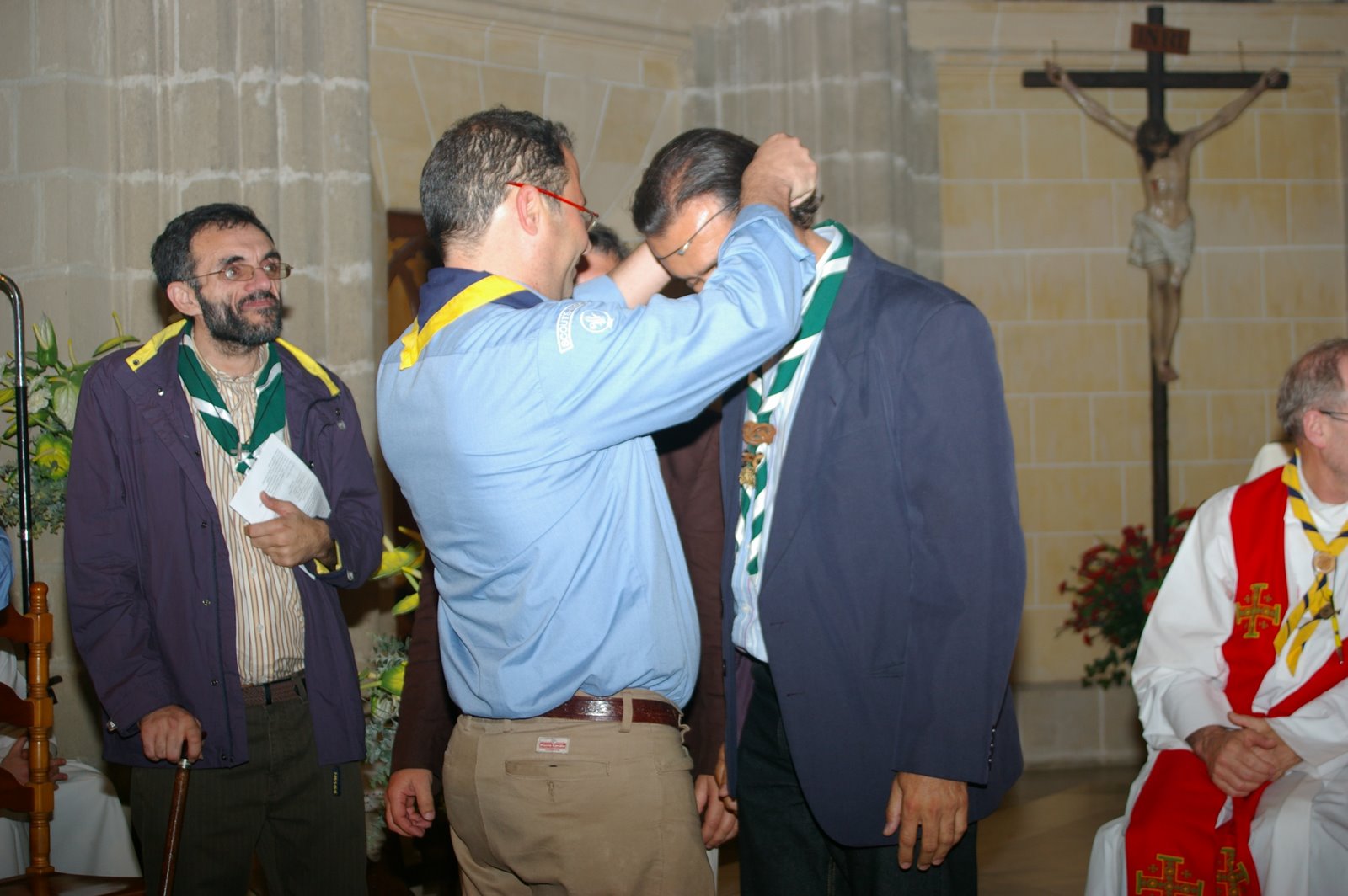In the image, a man in a dark blue coat with a green and white tie is bending his head down slightly to receive a medal from another man in a light blue shirt and khaki pants. The man giving the medal also wears a blue and white scarf. This ceremony takes place in a church, evidenced by the prominent crucifix with Jesus nailed to it on the right side of the image, accompanied by red and green flowers at the base. 

To their right, a priest, dressed in white robes with a red scarf featuring religious symbols, sits nearby, holding his hands together and looking in another direction. Another man in the background, leaning heavily on a cane and wearing a blue coat with a green and yellow scarf, holds some kind of document and observes the scene. The church's tan and gray walls form the backdrop of the image, giving a solemn and reverent atmosphere to this ceremonial moment.